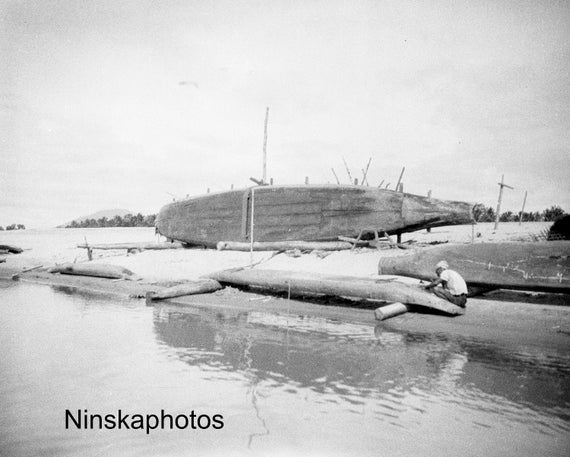This black-and-white photograph captures a detailed scene at a boat yard situated by a calm body of water. In the foreground, a man wearing blue jeans and a white shirt is squatting down, meticulously carving a long, slender wooden boat propped up on two logs; the smaller log supports the right end where he is working, while a larger log supports the other end. This boat appears to resemble a canoe. To the right of the man, slightly behind him, another smaller overturned boat is visible.

Dominating the background is a large, wide wooden boat turned on its side, revealing its flat bottom. The boat's shape tapers to a point on the right and is rounded at the left, supported by primitive scaffolding, including a log underneath for stabilization. A thick rope is tied around this boat, adding to the rustic charm of the scene. The shoreline is sandy, extending to a tree-lined horizon with sparse power poles visible. The sky is a blend of gray and white hues, contributing to the image's somber atmosphere.

In the bottom left corner of the photograph, the inscription "Ninska Photos" is clearly etched, underscoring the authenticity of this serene, labor-intensive moment captured along a tranquil beach.